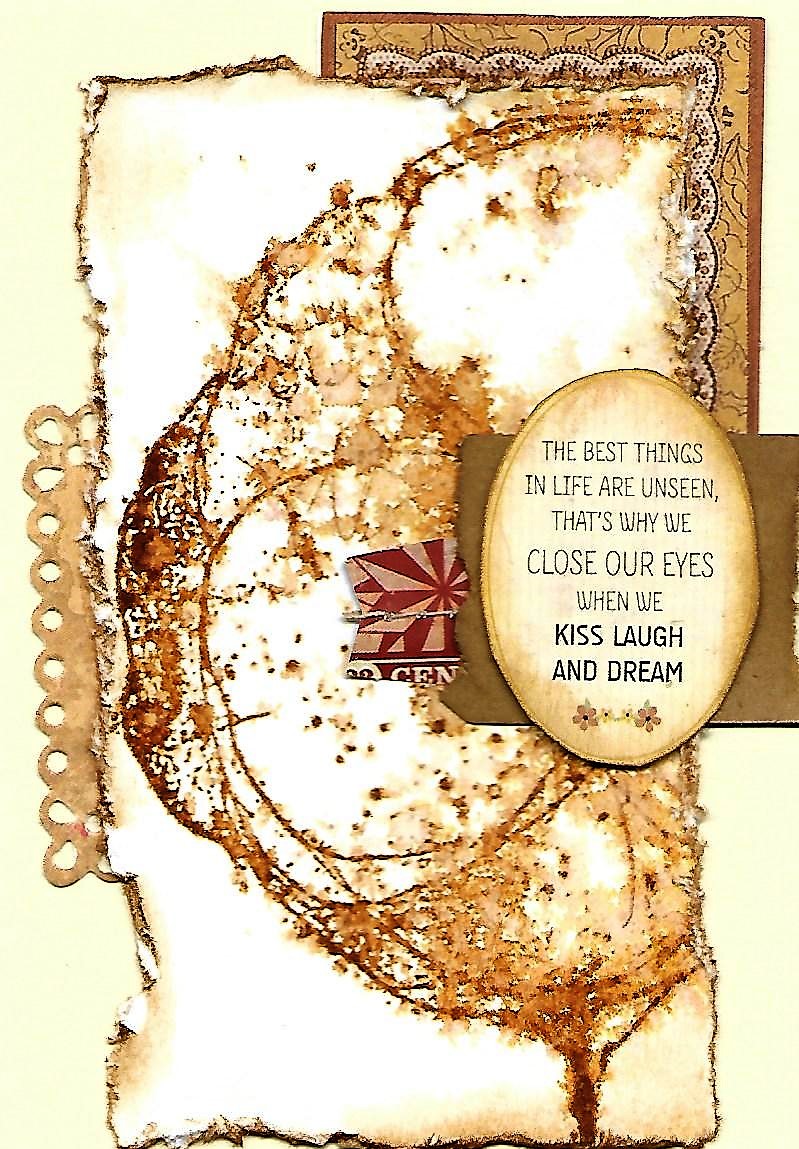The image features a meticulously crafted collage with a distinctly retro feel, utilizing aged and water-damaged elements for a textured appearance. The background is a mix of light brown and white, giving it a worn, vintage look. Central to the composition is a combination of used wood or tissue-like material. Layered atop this base is a prominent section of red and white paper arranged to resemble a pinwheel. 

Dominating the collage is a striking gold-embellished torn piece of white paper, creating a contrast against the rustic background. Further adding to the visual complexity, there's a half-circle of golden print etched onto the paper. Positioned to the right within the collage, an egg-shaped, oval piece of paper serves as a focal point. Beneath it lies a small, square fragment of torn paper.

Inside the oval, a poignant quote is elegantly inscribed: "The best things in life are unseen, that's why we close our eyes when we kiss, laugh, and dream." This thoughtful message is framed by the collage’s eclectic yet harmoniously arranged assortment of damaged, vintage elements, evoking a sense of nostalgia and romanticism.